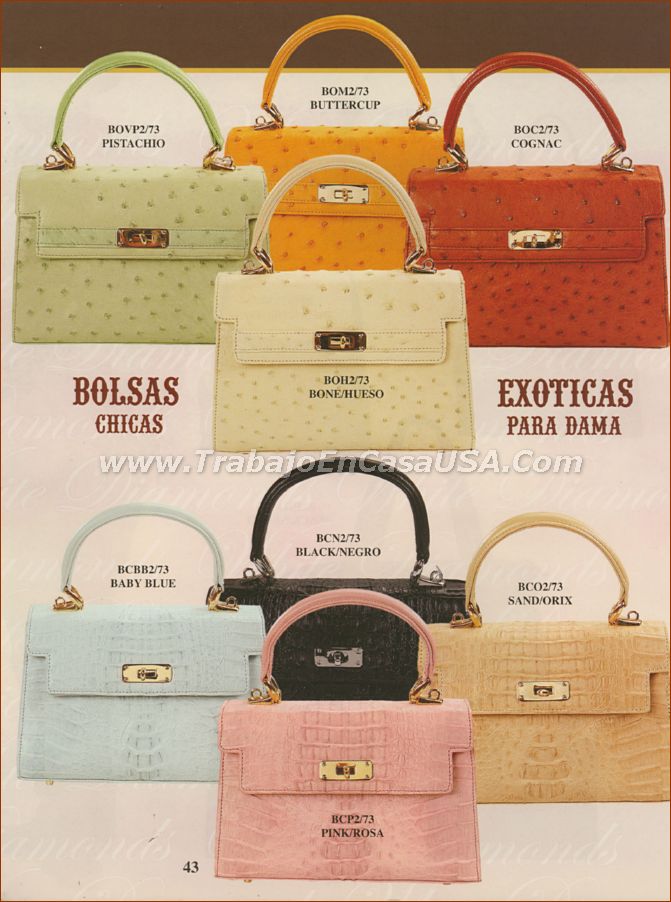The advertisement prominently features an elegant series of exotic designer handbags arranged in a visually appealing pattern. At the top of the image, there's a brown stripe followed by a narrow gold stripe spanning the width. Centered beneath this header is a striking assembly of four handbags: from left to right and slightly staggered, the colors are Pistachio (green), Buttercup (yellow), Bone (cream), and Cognac (orange). These bags feature a short loop handle designed for handheld carrying and are adorned with luxurious gold clasps and hardware.

The display is mirrored beneath the first set, presenting another four handbags in complementary shades: BB Blue (blue), Black, Sand (brown), and Pink. Each row of handbags forms a diagonal arrangement resembling a sideways diamond, reinforcing the stylish and symmetrical composition of the advertisement.

Further distinguishing the bags, the top set flaunts a sleek, dotted pattern, while the bottom set emulates a sophisticated alligator skin texture. The center-right of the image prominently features the brand name “Bolas Chicas” with the tagline "Exoticas Paradama" below it. The website, www.tabloidoenquesousa.com, appears in white text beneath the branding, directing viewers for more information or purchase. The harmonious arrangement and detailed textures emphasize the exquisite craftsmanship and diverse color palette, tempting viewers with a luxurious array of handbag options.